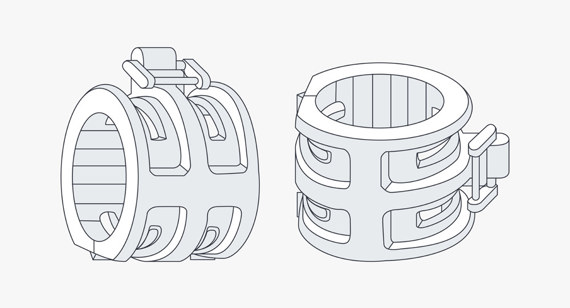This computer-rendered image features two cylindrical braces set against an off-white background, each highlighted in grey tones. Both braces, likely designed for industrial use, are identical and equipped with clamping mechanisms. The brace on the left is depicted horizontally, with its open end angled slightly forward, while the brace on the right is shown upright, resembling a cup set on a flat surface. Each brace displays four indentations along its sides and has a ridged interior, enhancing its grip. The detailed render showcases the clamps from different viewpoints, providing a comprehensive understanding of their structure and function.